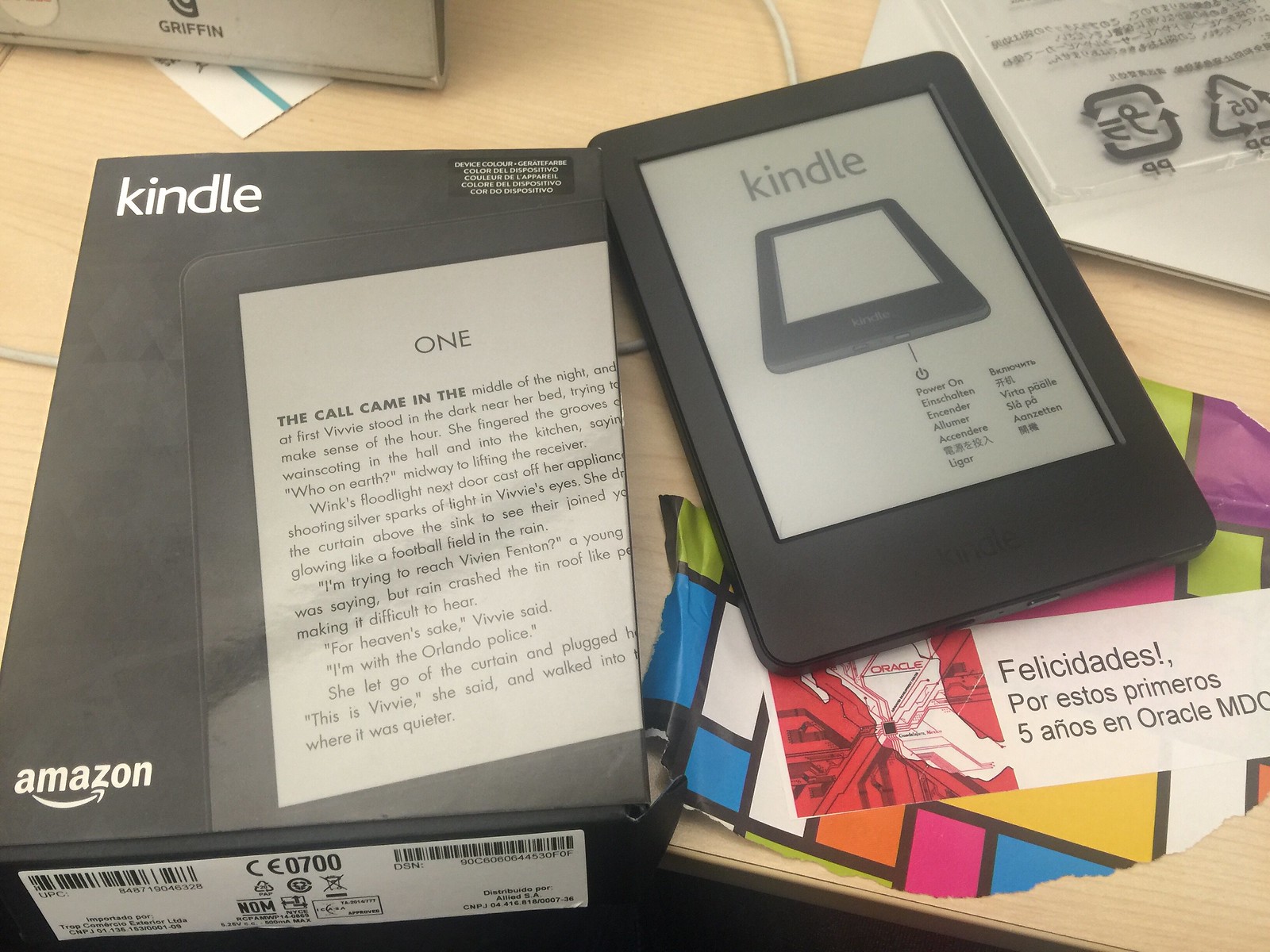The image captures a top-down view of an Amazon Kindle alongside its packaging, positioned on a light-colored, wood-grained table. The left side of the frame is dominated by the Kindle's black box, which features an image of the device displaying a Kindle screen, alongside multiple barcodes and product information at the bottom. The Kindle itself is on the right, its screen displaying the word "Kindle" at the top, an illustration of another Kindle, and what appears to be setup instructions. Below the Kindle, there is a piece of multi-colored wrapping paper and a note that reads, "Felicidades por estos primeros 5 años en Oracle MDO." The entire setup, inclusive of a few visible cords and edges of other papers or folders, suggests that the Kindle is a recent gift placed carefully next to its package.